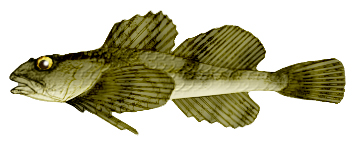The image is a detailed illustration of a green fish, generated using a computer program. The fish is depicted from a side view, showcasing a slightly open mouth, one visible eye, and several fins. The eye is yellow with a black pupil and a hint of white. The fish's body has a greenish hue mixed with pops of black and white highlights, and the scales are visibly detailed along its back. The fins are olive green with striped patterns, and the fish has a total of five fins along with its tail fin. The head of the fish is larger than its tail, which is positioned towards the right side of the image, while the head points to the left. The background is stark white, providing no indication of water, making the fish appear as if it’s suspended in midair. The overall focus of the illustration is on the fish's serene, slightly mopey expression, and its aesthetic details, set against a minimalistic backdrop that emphasizes its features.